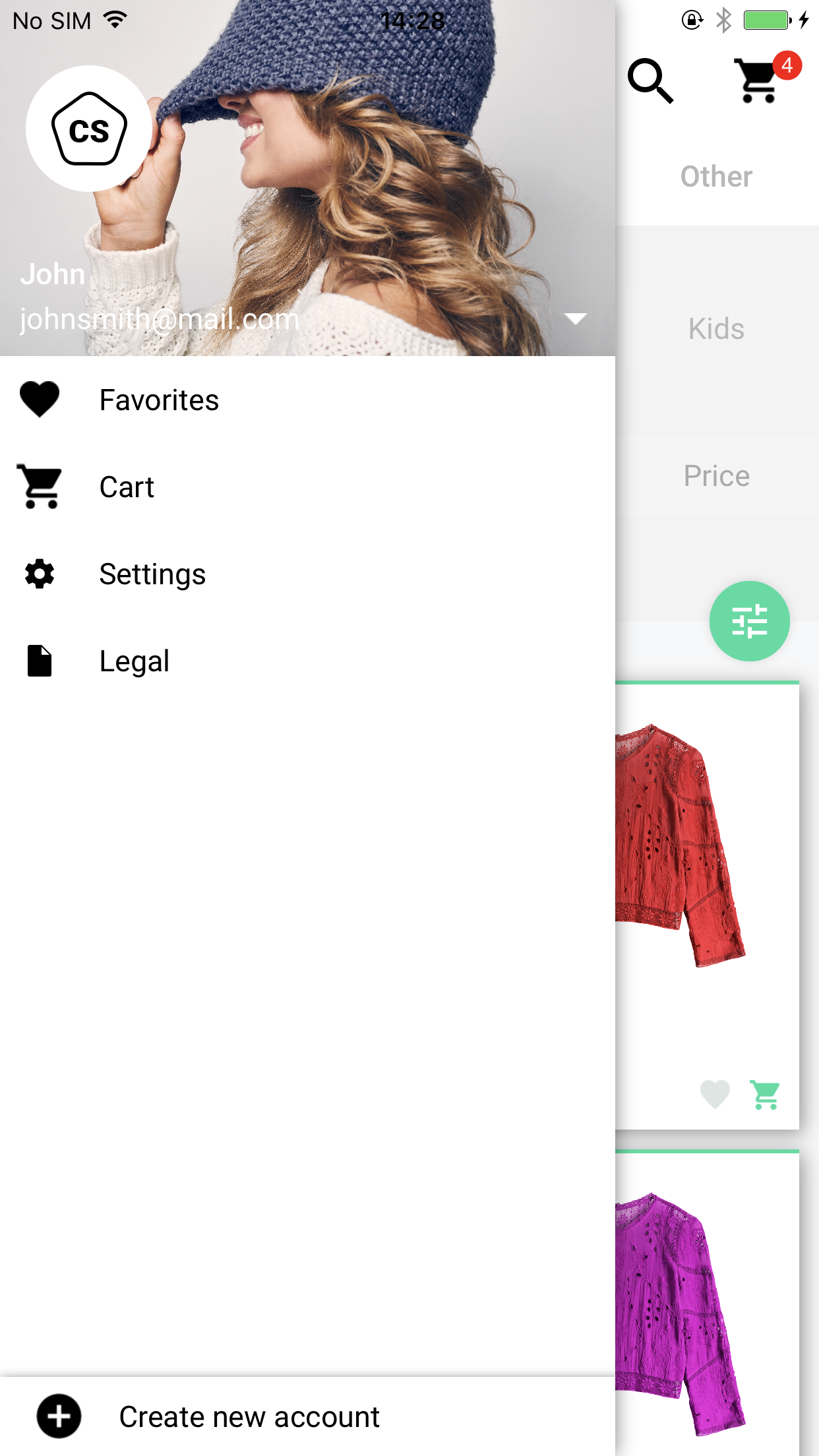The screenshot showcases a shopping app, prominently featuring an expanded menu on the left side that occupies the majority of the screen. At the top of this menu is an image of a smiling white woman in profile view. She is wearing a beanie pulled down over her nose, a white sweater, and has blonde curly hair.

Superimposed on the woman's image is a white circle containing a pentagon with the letters "CS" within it. Adjacent to the circle is the text "John," followed by "JohnSmith at mail.com."

Below this, the menu area is predominantly white and includes multiple options: 
- "Favorites," accompanied by a heart icon 
- "Cart," accompanied by a shopping cart icon
- "Settings," accompanied by a gear icon
- "Legal," accompanied by a document icon

Beneath these menu options is a significant amount of white space, followed by two buttons: a plus sign option and "Create New Account" at the bottom of the menu.

In the portion of the screen not covered by the menu, a red notification circle with the number four inside appears over a shopping cart icon in the top-right corner. Below this, partially visible, are options related to different price categories for kids and snapshots of items available for purchase, including a women's red sweater and a green or purple sweater.